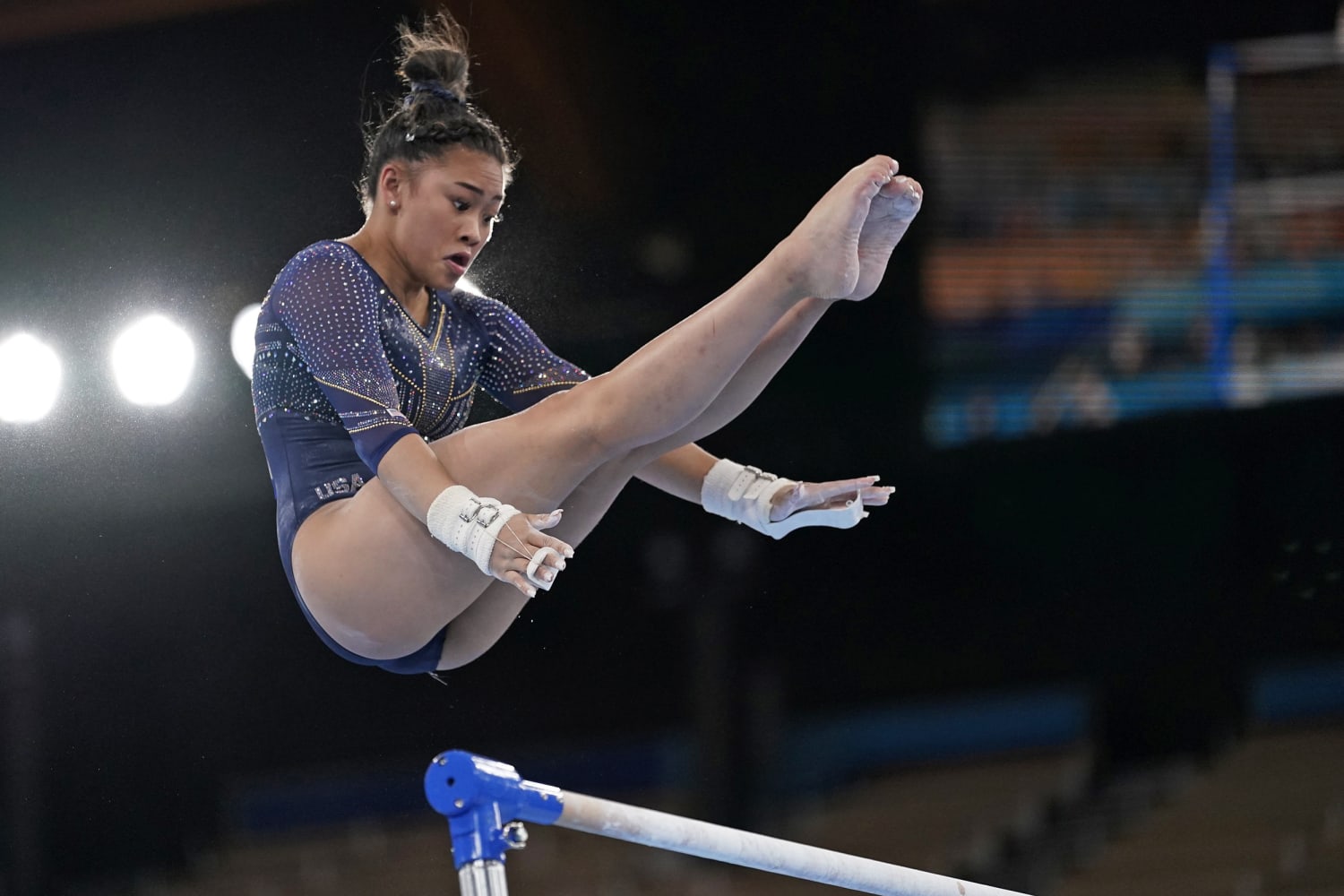This color photograph captures an action shot of a young female gymnast performing a trick off the uneven bars. She is in mid-air with her body bent into a V shape, legs straight out in front of her and toes curled. Her hands reach toward the white, powder-dusted bar beneath her, which has blue end caps. The gymnast is wearing a blue, sparkly bodysuit adorned with crystals that spell out "USA" above her thigh. She has leather gloves with two straps that act as grips for the bar, and her wrists are wrapped in white tape with additional tape on her fingers. Her dark hair is tightly secured in a bun on top of her head. The background showcases a blurred arena with three spotlights and indistinct seat silhouettes, suggesting an empty or sparsely populated venue.